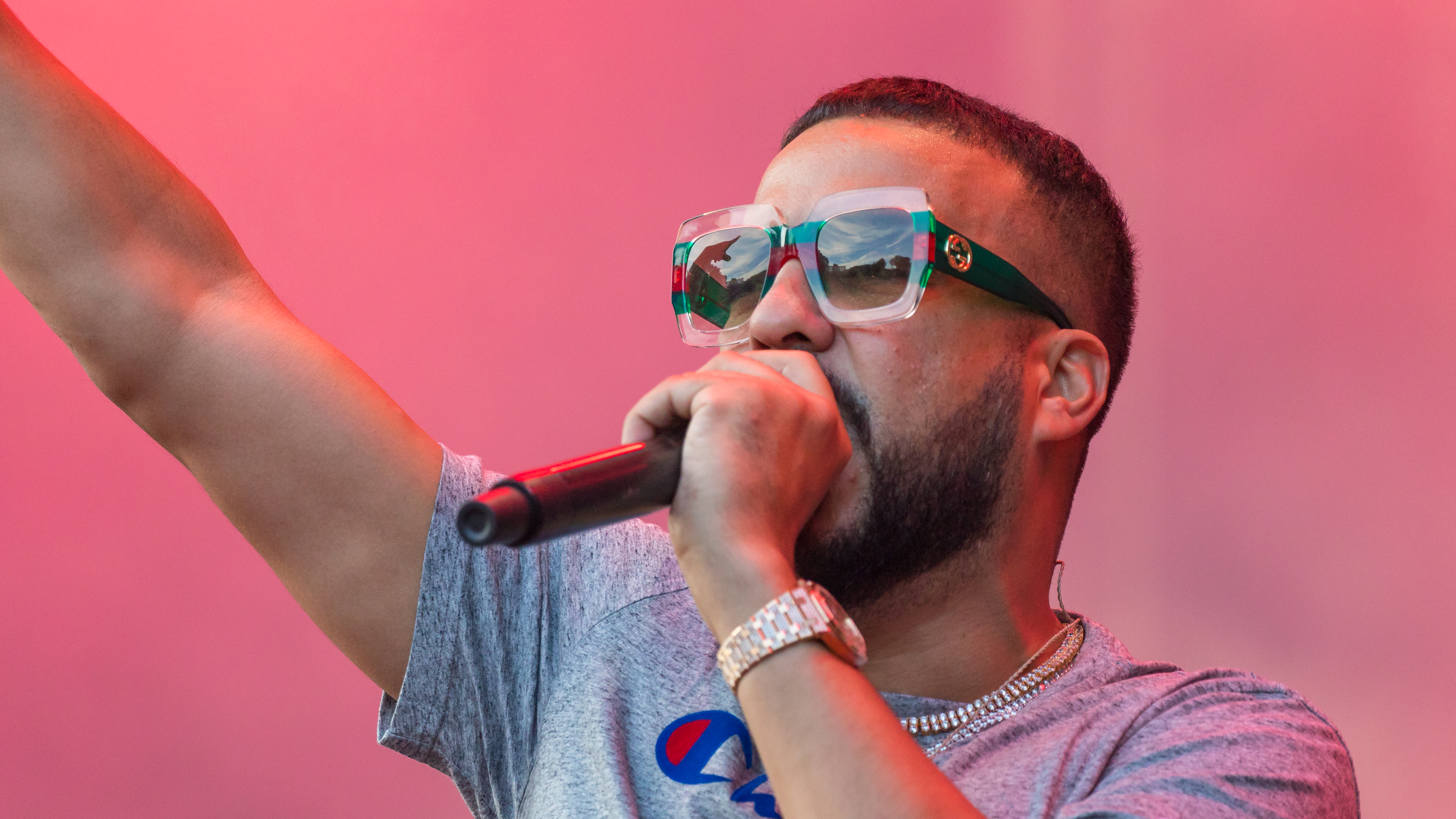This image depicts an African-American male, likely a rapper or singer, performing against a striking pink background that fades to a lighter hue on the right. The man, visible from the shoulders up, has light brown skin, short dark hair, and a full dark beard that is longer than the hair on his head. He is wearing vibrant sunglasses that are green, red, and clear with a gold logo. His gray short sleeve t-shirt features a symbol resembling a blue 'C' with red detail, possibly the Champion emblem. Around his neck are two gold chains, and on his left wrist, he sports a gold watch. In his left hand, held close to his mouth, is a black microphone. His right arm extends at a raised angle towards the top left corner of the image, cut off halfway down the forearm.